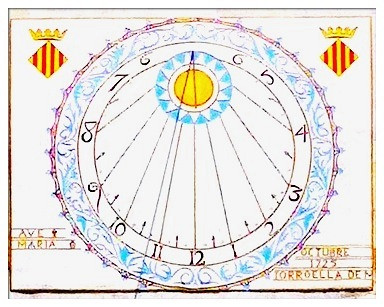This is a detailed sketch with elements that suggest a vintage clock or sundial appearing to be taken from an old book. The artwork, resembling a crayon drawing on a white background, features a large central circular dial outlined in purple, surrounded by a blue floral border. The dial is detailed with numbers from 1 to 12, arranged clockwise, and intersected by diagonal lines pointing towards the dial's center, which interestingly is not located centrally but rather at the top.

At the top center between the 6 and 5, there is a vibrant depiction of a sun with a yellow center, encircled by a thin red line and a blue outer ring adorned with about 20 white rays. Adjacent to this central sun icon, there is notable text: "Ave Maria" written on the bottom left, and "October 1725, Torella D.E.M." inscribed on the bottom right.

In both the top left and top right corners of the sketch, identical diamond-shaped emblems are presented. These diamonds are decorated with red and yellow horizontal stripes and are topped with gold crowns, adding a regal touch to the image. The entire composition gives the impression of an intricately designed, old-fashioned timekeeper, combining artistic and historical elements seamlessly.